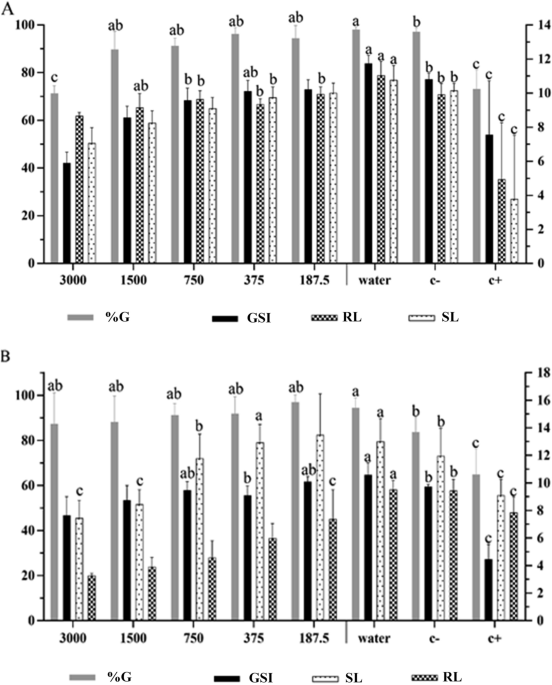The image displays two bar charts, one positioned at the top and the other at the bottom, both featuring light gray and black bars. Each chart is marked with the labels A and B and includes tiny bar segments labeled with a series of repeated letters such as C, A, and B. The left side of each chart's y-axis is numbered with intervals reaching up to 100, while the right side has intervals reaching from 0 to 18. Additionally, another axis is labeled with larger numerical values like 3,000 and 1,500. Both charts appear to have a consistent labeling system involving GSI denoting a bold black line, RL represented as a black and white checkerboard, and SL depicted as a dotted white line. These elements are mirrored across both the top and bottom charts, contributing to an intricate and detailed visualization of the data presented.